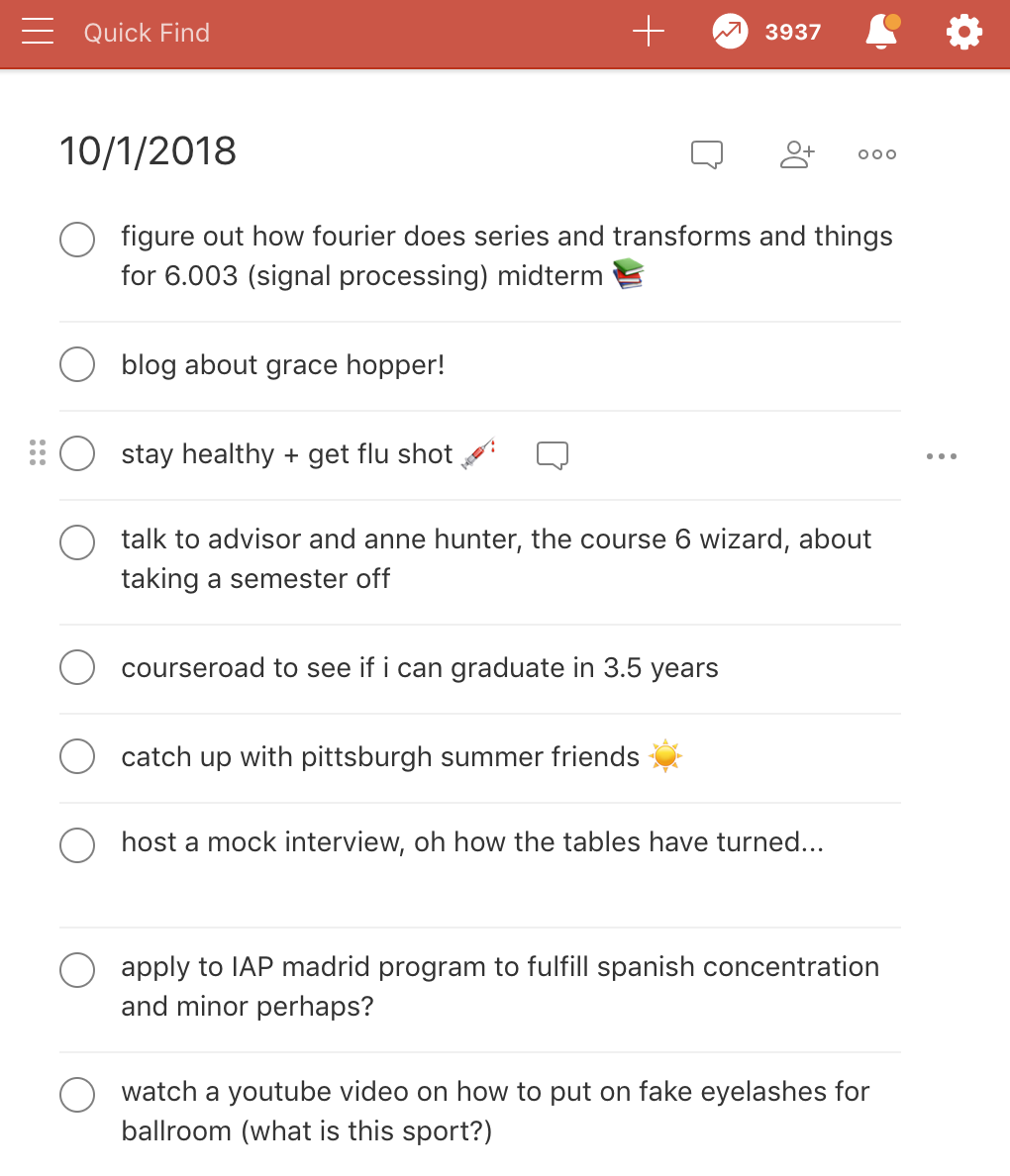The image depicts a screen capture of an online application interface. At the top, a red horizontal bar features several elements. On the left side of the bar, the words "Quick Find" are written in white. On the right side, there is a sequence of icons: a white plus sign, a red jagged arrow contained within a white circle, the numerals "3937," an alarm icon, and a settings icon represented by a circular gear.

Beneath this red bar, the date "10-1-2018" is displayed on the left. On the right side, there are three icons: a call-out bubble, a person silhouette, and a set of three dots indicating a menu or additional options. 

Below the icons and date, the main body of the screen shows a list of bullet points in black text. The first bullet point reads: "Figure out how Fourier does series and transforms and things for 6.003 Signal Processing Mid Term."